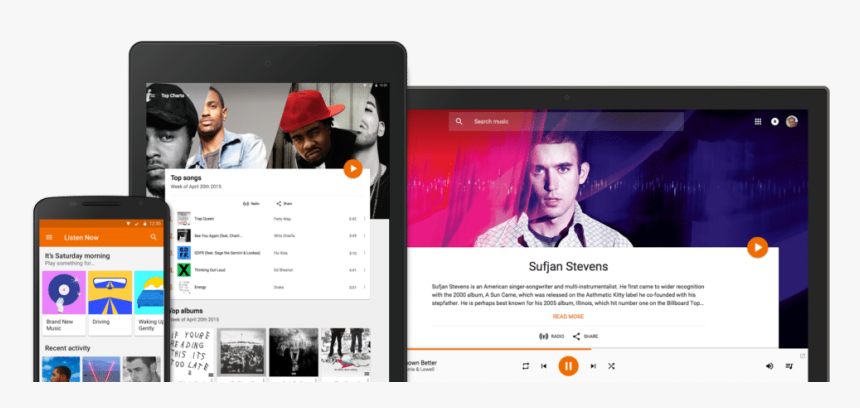This digital image showcases a variety of electronic devices, including a cell phone, a tablet, and a laptop, each with their screens illuminated. The focus is on the cell phone screen, which prominently displays a "Listen Now" option accompanied by the message, "It's Saturday morning, play something for brand new music." Below this, various curated playlists are featured with descriptive images: one titled "Driving" shows a road and a rearview mirror, another titled "Waking Up Gently" displays a bed with a headboard. Additionally, there are multiple images on the cell phone screen, including singers, the artist Drake, and an African American man wearing a red hat sideways. The titles of the top songs are visible but blurry. The laptop screen in the background shows a clear picture of a man, appearing to be around 27 years old. The tablet is also powered on, adding to the array of gadgets depicted in this image.